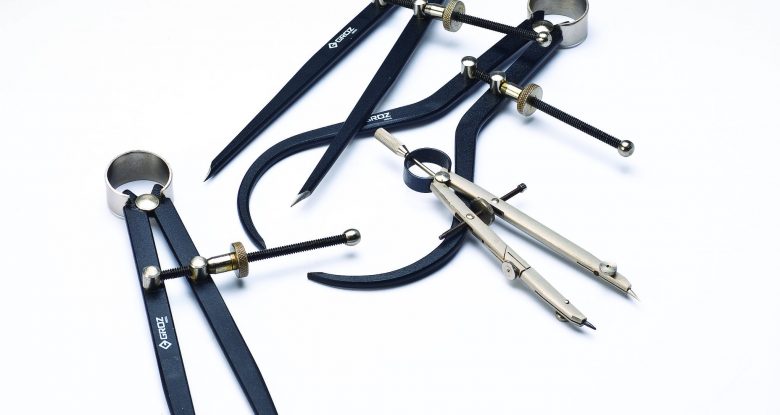The image features a variety of compasses, typically used for drawing circular shapes with a pencil, displayed on a white background. In the bottom right corner, there is a classic silver compass, characterized by two long, thin, silver legs joined at the top. This compass includes an adjustable mechanism to change the width between the legs, allowing for different circle sizes, and ends in sharp points.

To the left, there is a black compass, and another black one in the upper right corner. Additionally, in the upper right, there is a tool resembling a caliper, possibly intended for measuring body fat. This caliper-like instrument is distinct with its rounder base where the legs join together, in contrast to the more traditional compass designs. All these tools feature tighteners in the middle for adjusting the span and have sharp points at the ends to anchor and create precise circles. The instruments have tags indicating their brands, though the labels are difficult to read in the image.